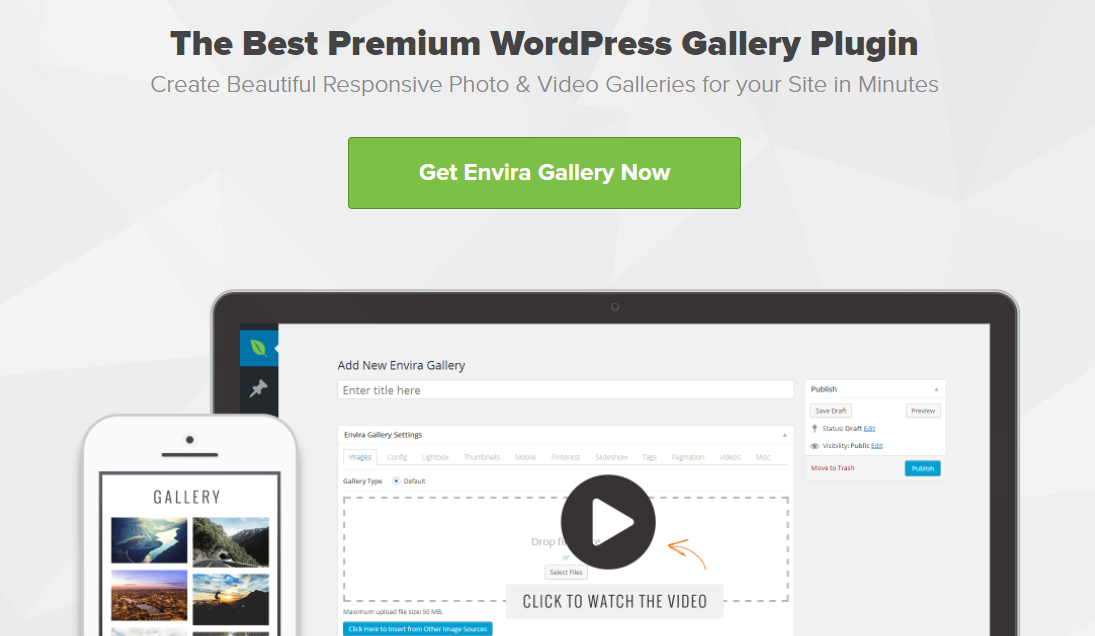The image is a left-to-right horizontal advertisement layout with a gray background showcasing a range of geometric shapes in various shades of gray, adding subtle dimension without noticeable texture. At the top, prominently displayed in bold black text, is the headline: "The Best Premium WordPress Gallery Plugin." Below this, in slightly less bold black text, is the subheading: "Create beautiful responsive photo and video galleries for your site in minutes."

A green rectangular button stands out with white text, inviting users to "Get EnviroGallery Now."

To visually represent the product, partially visible images of a smartphone and a tablet or computer are included. The white smartphone features a single black-lined camera and displays an example gallery with landscape photos. The tablet or computer, distinguished by its black border, shows an open EnviroGallery interface. The interface includes a gray pop-up box labeled "Add New EnviroGallery," where users can enter a title and access settings. There is also a play button available to watch a tutorial video. To the right side of this interface is another smaller box with options to publish, save drafts, or preview the gallery, providing additional information and controls for users.

This comprehensive display effectively highlights the features and functionality of the EnviroGallery plugin, appealing to potential users looking for an easy and responsive gallery solution for their websites.